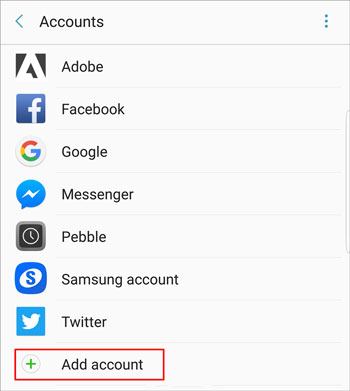The image features a vertically-oriented white rectangle bordered by a thin gray line. At the top of this rectangle, a heading titled "Accounts" is highlighted with a left-pointing arrow, setting it apart from the rest of the text, which is left-justified. Beneath this heading runs a faint gray line, separating it from the subsequent list of items.

Each item in the list is preceded by a respective logo and the items are separated by faint gray lines. The listed accounts are as follows: Adobe, Facebook, Google, Messenger, Pebble, Samsung, and Twitter. At the bottom of this list, there is a green plus icon followed by the text "Add account" in black, all enclosed within a red-rectangle border, suggesting a focal point for initiating the addition of new accounts.

The predominant colors in the image are black, white, gray, with accents of blue, red, yellow, and green, indicating a visually-coded instructional design. The red border around the "Add account" section implies the image's use for educational purposes, likely illustrating how to add accounts on a device.

In summary, the image appears to serve an educational purpose by guiding users on how to manage and add their accounts, using color coding and clear demarcations for instructional clarity.